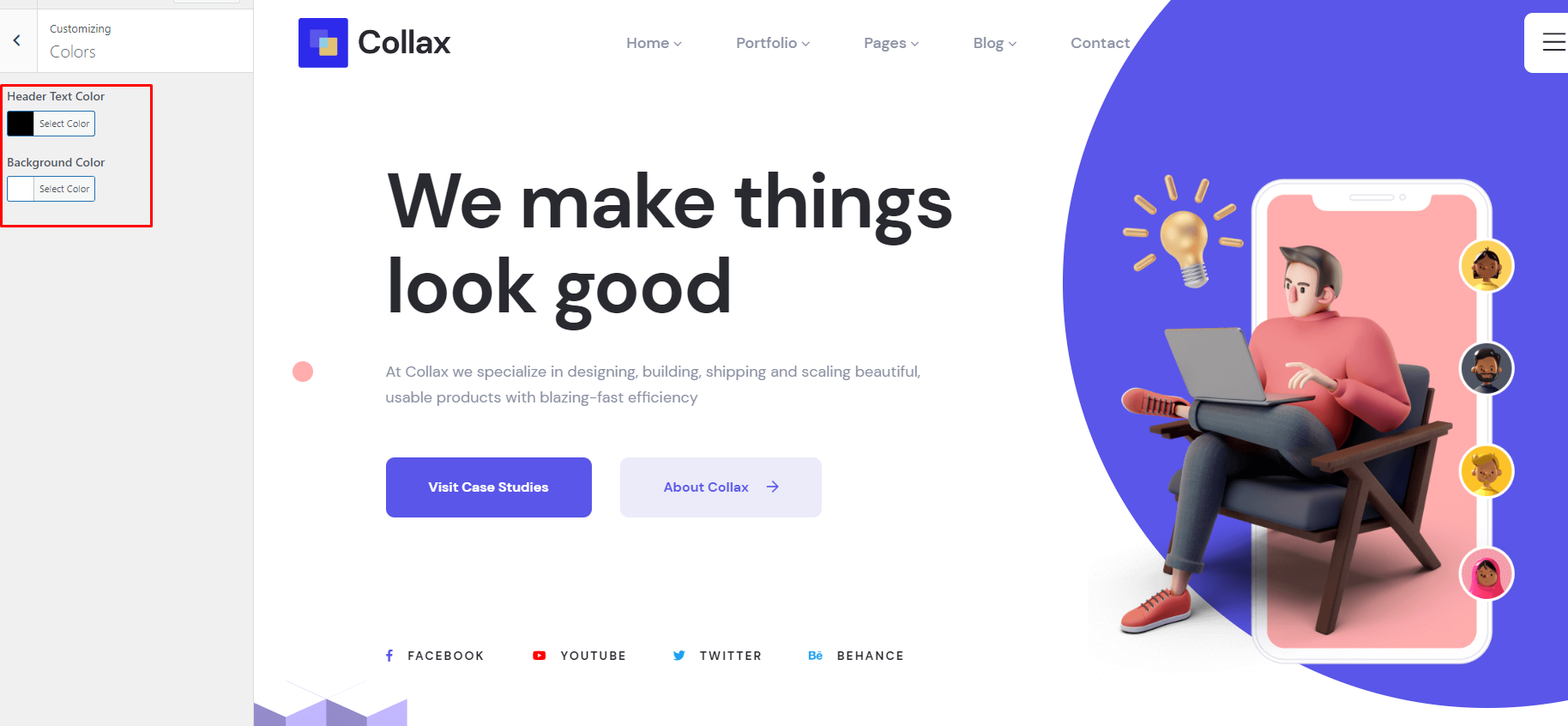The image showcases a web page from a website named "Colax." On the far left of the interface, there are customization options prominently displayed. These include sections for adjusting the color scheme with options such as "Header Text Color," which shows a black square alongside a "Select Color" prompt, and "Background Color," where a white square appears with the option to "Insert Color or Select Color."

Moving to the central part of the design, the web page features the Colax logo, a large blue square with smaller squares in the upper left corner, alongside the brand name "Colax" in capital letters (C-O-L-A-X). Below the logo is the primary navigation menu, which includes buttons labeled "Home," "Portfolio," "Pages," "Dialog," and "Contact."

On the right side of the web page is a prominent column containing an animated graphic. This graphic depicts a generic cell phone with an animated person sitting on a living room chair, legs crossed, working on a laptop, with a light bulb icon above them. Adjacent to the cell phone graphic, there are four circular profile pictures displayed.

In the middle section of the web page, a bold statement reads "We Make Things Look Good," followed by two call-to-action buttons: "Visit Case Studies" and "About Colax."